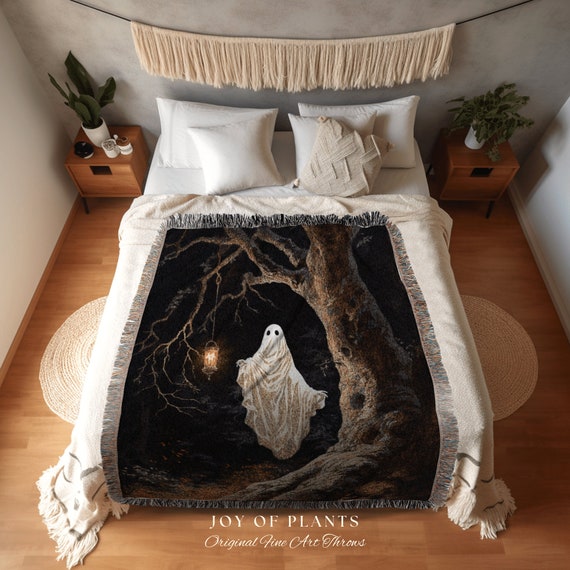In this detailed image captured from an above view, a white double bed dominates the center against a backdrop of light brown wooden flooring and off-white walls. The bed is neatly made, featuring a white blanket and four white pillows, two on each side, complemented by a textured tan pillow with zigzag patterns, slightly tilted to the right. A smaller, intricately designed blanket, fringed at the edges, adorns the center of the bed, displaying a dark nighttime scene with a ghost draped in a white sheet, eyes peeking through, floating beneath the barren branches of a craggy tree. The tree's thick, gnarled trunk and lifeless branches stretch across the right side of the image, supporting a hanging lantern to the left of the ghost. Flanking the bed are two wooden nightstands, each housing a green plant in a white flower pot, resembling file cabinets with drawers. Above the head of the bed, a decorative banner made of delicate, hanging strings adds a touch of whimsy to the room. At the foot of the bed, the inscription "JOY OF PLANTS" in bold, all-caps text, followed by "original fine art" in smaller, italicized letters, completes the serene and slightly eerie scene.